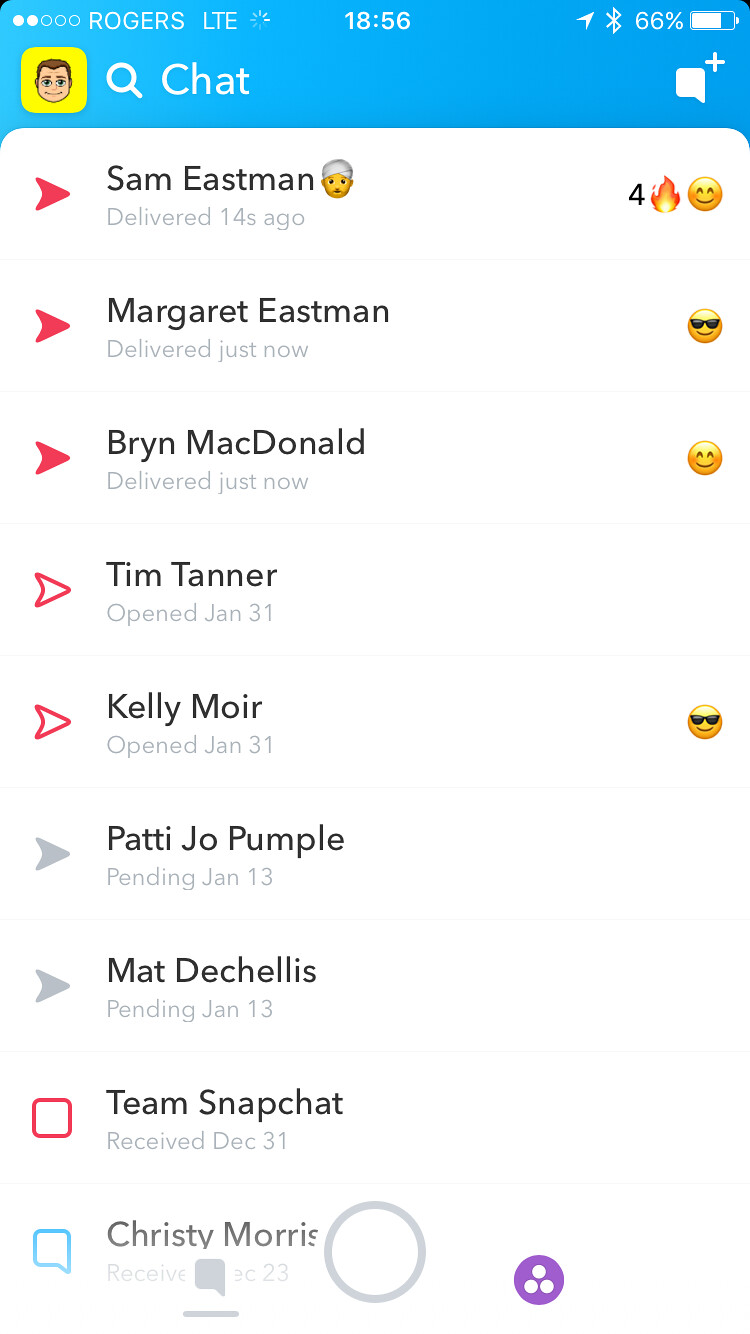The image is a rectangular screenshot of a Snapchat chat log taken from a smartphone. Dominating the upper left corner is the cell provider name, Rogers LTE, and adjacent to it at the top center is the time displayed as 18:56. The phone’s battery life stands at 66%, easily visible in the status bar. Below this, a blue banner stretches across the screen, including a yellow square icon featuring a cartoonish man's face, a search bar, and the word "chat." The chat list starts right beneath this bar, displaying the names of people engaged in conversation: Sam Eastman, Margaret Eastman, Bryn MacDonald, Tim Tanner, Kelly Moore, Patti Jo Pumple, Matt Deshilis, Team Snapchat, and Christy Morris. To the right of some names, there are various emojis, including a fire emoji, a smiley face, and a smiley face with sunglasses.